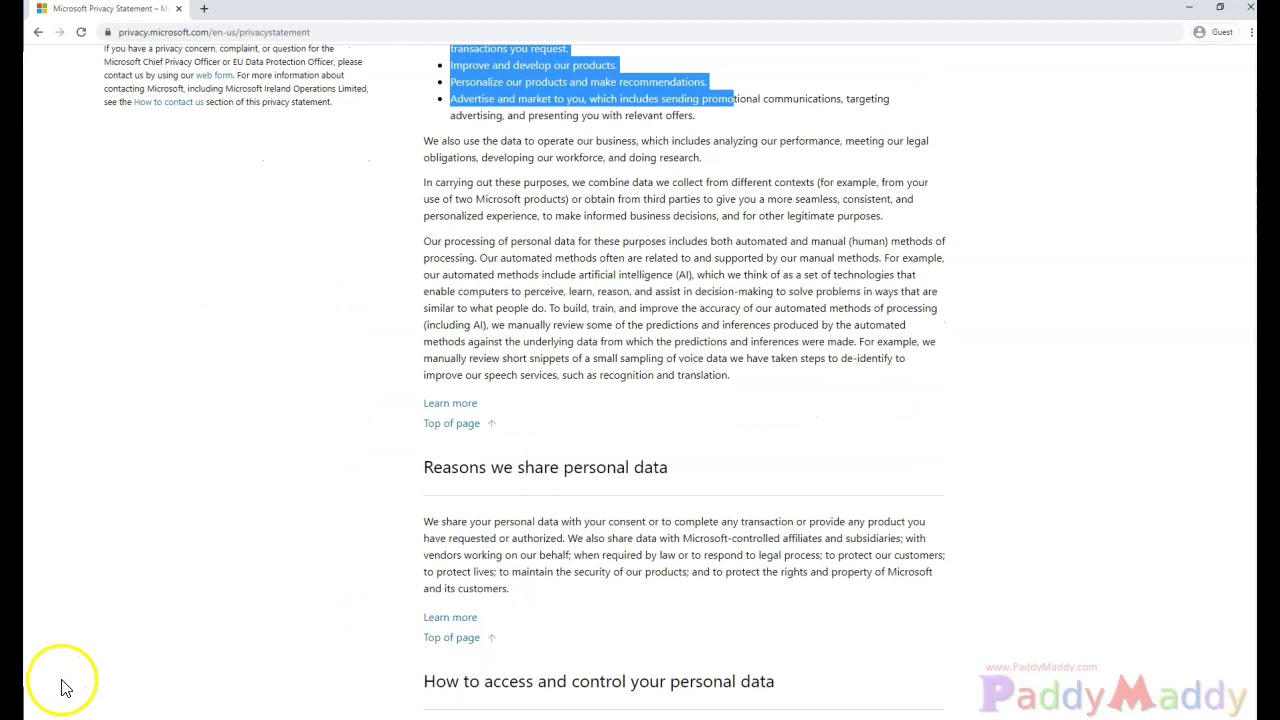A detailed screenshot of the Microsoft Privacy Statement webpage is displayed. At the top, there's a browser tab open with the title "Microsoft Privacy Statement" in gray font accompanied by the Microsoft icon to its left. Just beneath this, a URL bar shows the web address "privacy.microsoft.com/en-us/privacy-statement." The screenshot captures the entire page, which comprises the privacy statement text.

The text explains, "We also use the data to operate our business, which includes analyzing our performance, meeting our legal obligations, developing our workforce, and conducting research. In carrying out these purposes, we combine data collected from different contexts — for example, from your use of two different Microsoft products or data obtained from third parties. This integration aims to provide a more seamless, consistent, and personalized experience, enable informed business decisions, and support other legitimate purposes. Our processing of personal data for these purposes includes both automated and manual methods. Often, our automated methods are related to and supported by our manual methods."